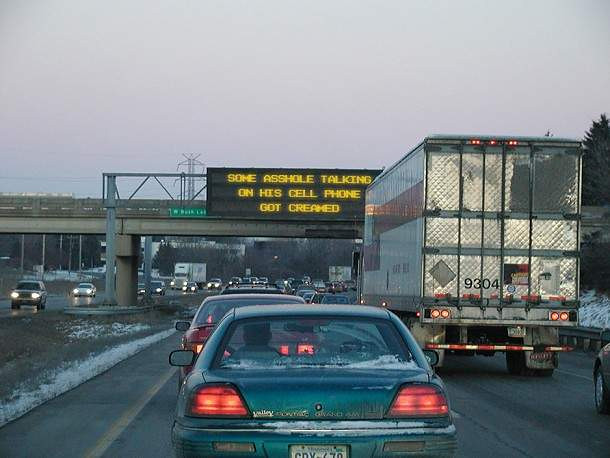A cloudy day sets a somber mood over a bustling street scene. In the foreground, the backs of several cars are visible, including a green sedan closely tailing a red compact car. The two sedans are driving on a main road, with a larger white truck occupying the far right side. Above the scene is a low highway bridge crossing the street. Attached to it is a prominent black sign with striking yellow letters that read, "Some asshole talking on his cell phone got creamed." On the left side of the image, another street merges with the main road, and it's filled with oncoming traffic, the headlights of numerous vehicles glowing through the dim atmosphere. The entire scene captures the hurried pace of city life under a blanket of overcast skies.